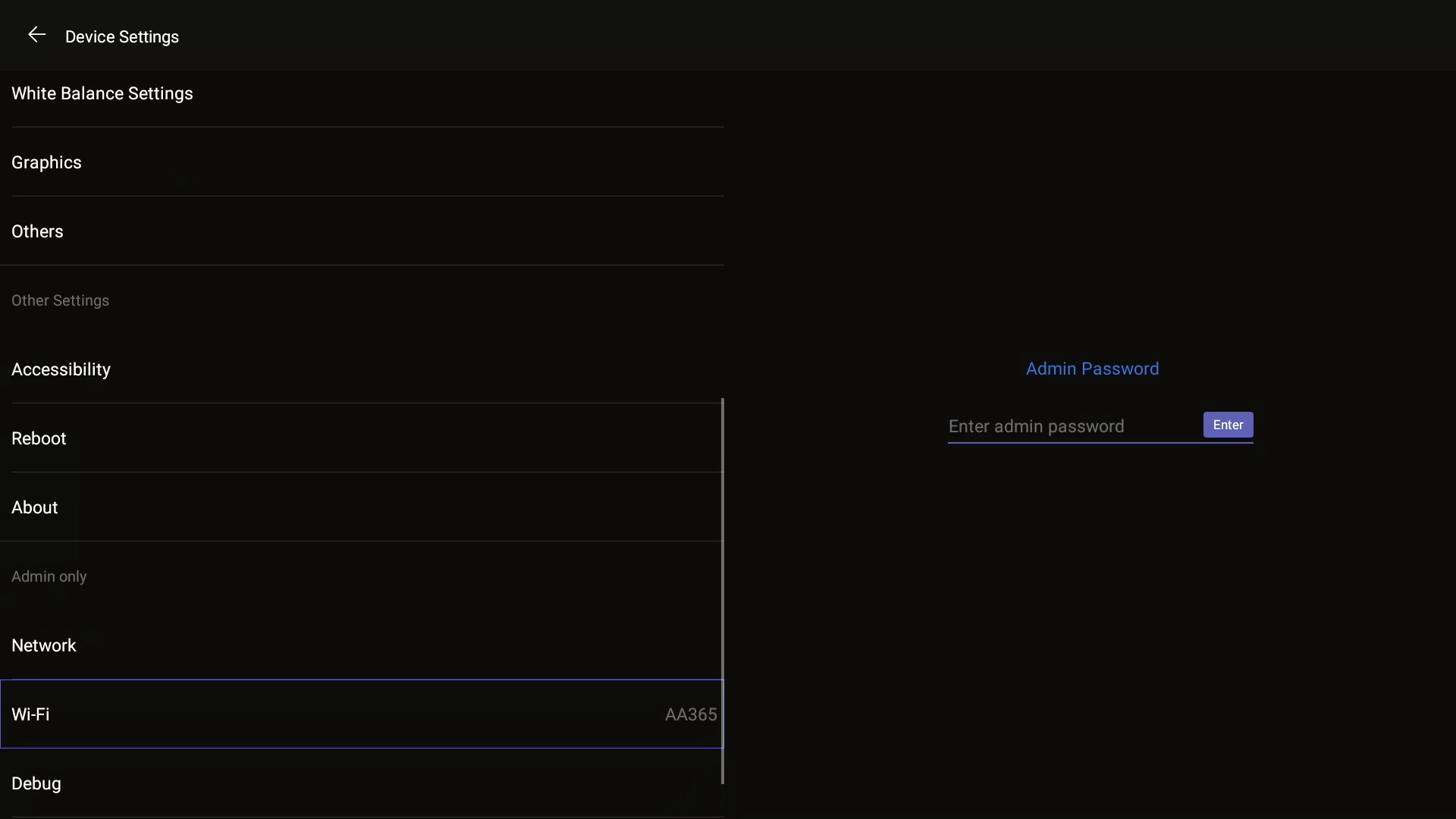In this image, the black screen is divided into two distinct sections: one on the left and one on the right. The left side features a white font listing various settings categories, each separated by a light grey line. Starting from the top, the categories include:
- A leftward arrow followed by "Device settings"
- "White Balance Settings"
- "Graphics"
- "Others," which is marked by a lighter grey font as "Other settings"
- "Accessibility" below which appear additional categories like "Reboot," "About," and “Admin Only"
- "Network," which includes a sub-category "WiFi" with the detail "AA365" indicated beside it
- "Debug"

On the right side of the screen, which is still black, a white line rises up to about halfway. Around the middle of this right section, blue text states "Admin Password," which is followed by a grey font instructing "Enter Admin Password." To the right of this text, there is a blue-purple button labeled "Enter" in white lettering. Just beneath this button, a purple line runs horizontally.

Overall, the image conveys a menu interface for device settings with a primary focus on administrative options.